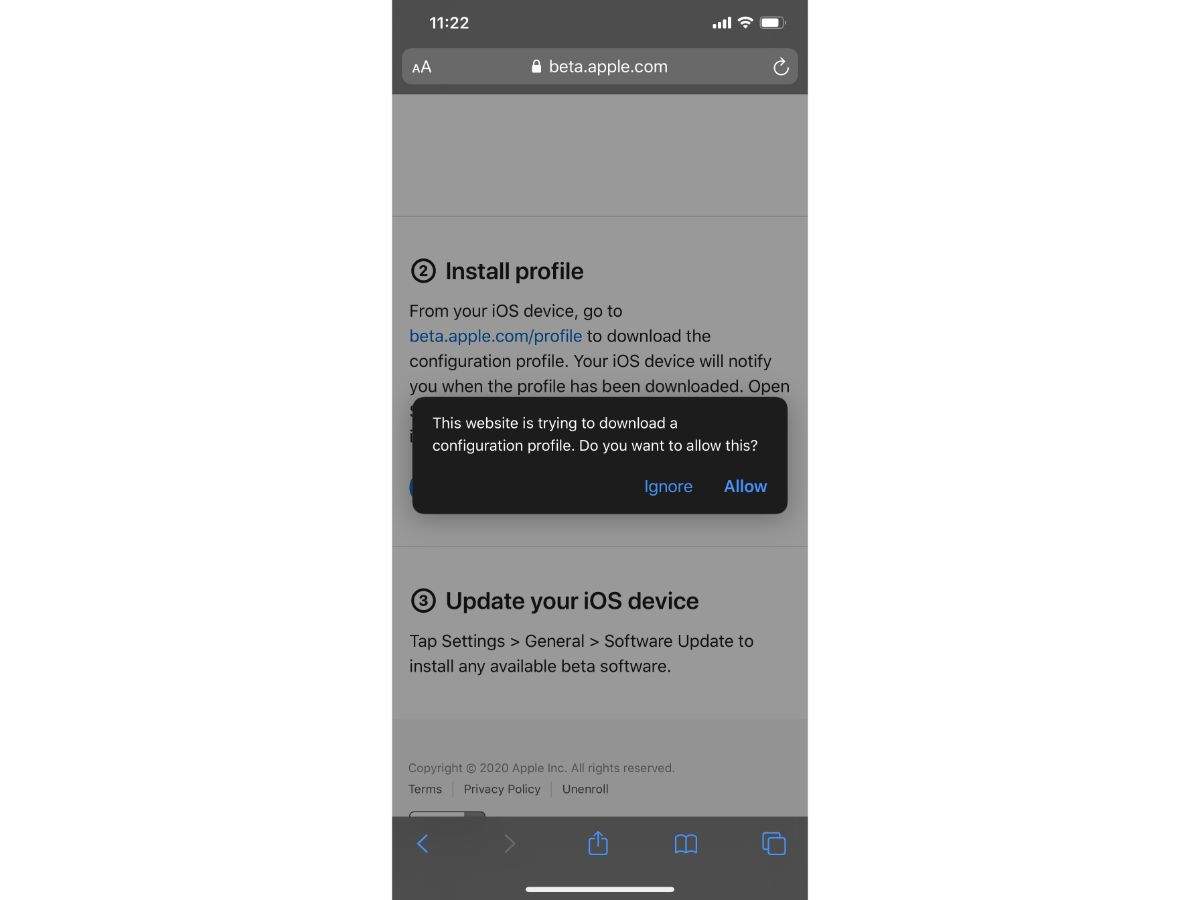**Caption:**

The image depicts an Apple iPhone displaying the Safari web browser on the website beta.apple.com. The device shows a time of 11:22 in the upper left-hand corner and full signal strength with four out of four bars and a complete Wi-Fi connection in the upper right-hand corner. The battery indicator indicates a nearly full charge.

The main focus of the screen is a pop-up dialog box prompting the user to either "Ignore" or "Allow" the download of a configuration profile. This prompt is displayed in a white box, with "Ignore" and "Allow" written in blue text, rendering the rest of the screen slightly grayed out until a choice is made.

Behind the dialog box, there is a series of instructions from the beta.apple.com website, guiding users on how to install a configuration profile on their iOS device. The visible steps include:

**2.** Navigate to beta.apple.com/profile to download the configuration profile. Your iOS device will notify you when the profile has been downloaded.

The third step partially visible:

**3.** Update your iOS device by accessing Settings > General > Software Update to install any available beta software.

Toward the bottom of the screen, the webpage displays links to Terms, Privacy Policy, Unenroll, and copyright information (Copyright 2020 Apple Inc., All rights reserved). Below these links, there are icons for navigating backwards and forwards, sharing, adding to favorites, and managing tabs in the Safari browser.